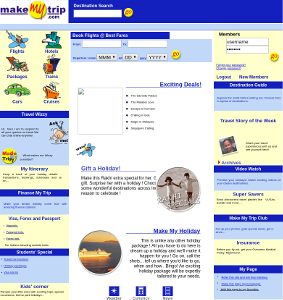Screenshot of a travel website interface on a white background. At the center top of the screenshot, there is a blue header featuring a white search bar. To the left of the search bar, there are several small icons representing different travel categories, such as flights, hotels, packages, rental cars, and cruises. These categories are indicated with small images, though the details are somewhat indistinct due to the image size. Some icons are marked with a blue color, others with red, and a yellow circle is also present.

The main body of the screenshot is divided into three columns. The left and right columns each contain blue rectangles with a dark blue header, and the right column has a section titled "My Pages," which includes three blue links and one black link.

In the middle column, there is a form with three input boxes labeled "MM" for month, "DD" for day, and "YYYY" for year. Below this form, a section titled "Exciting Deals" lists various promotional offers. Additionally, another section highlights specific deals related to holidays and gifts. The arrangement and color scheme emphasize a user-friendly interface aimed at aiding travel planning.